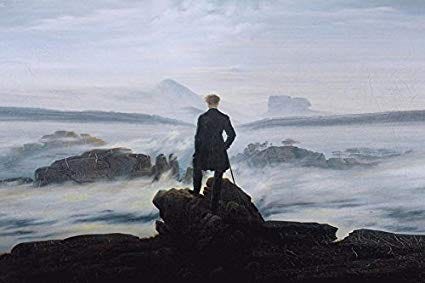This is an incredibly detailed and atmospheric image of a man standing on rocky bluffs beside a turbulent sea. The man, dressed in a long black coat and a distinctive hat – perhaps a top hat or a cap – stands poised with a cane in hand. The sea, mirroring the grays and whites of the overcast sky, thrashes against the rocks at his feet. Behind him, mountainous rocks rise at the horizon, creating a stark and dramatic backdrop. The overall scene, rendered in black and white, conveys a timeless sense of solitude and contemplation, capturing the man as he gazes over the dark, wave-crashed waters below. The clouds are a blend of white and gray, blending seamlessly with the shades of the ocean, adding an element of continuity and depth to the painting. The artist's talent shines through in the meticulous detail and the evocative mood of the composition.